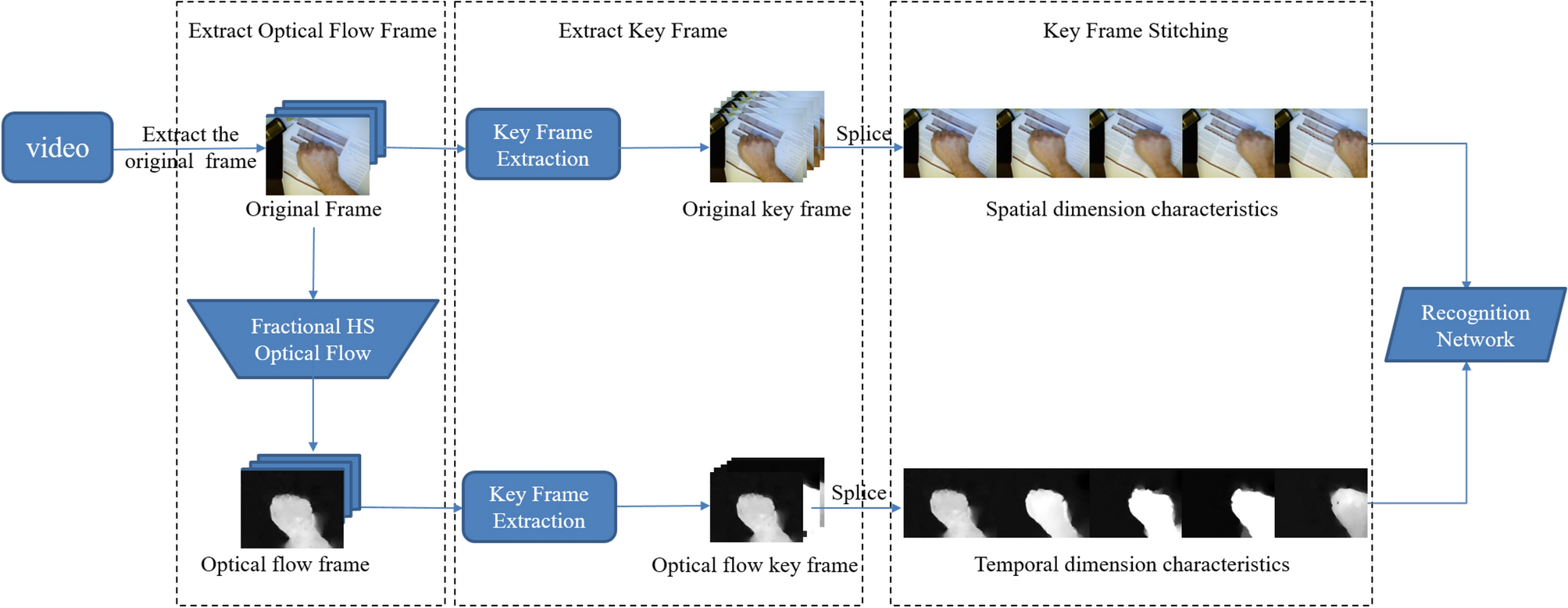This image presents a detailed flowchart depicting a complex process. Starting from the left, a blue rounded rectangle labeled "Video" leads via a blue arrow with the text "Extract the original frame" to an image representing the "Original Frame." This original frame flows into a panel titled "Extract Optical Flow Frame," showing an arrow descending to a blue trapezoid labeled "Fractional HS Optical Flow," and further downward to an "Optical Flow Frame" image. Simultaneously, an arrow extends to the right from the original frame into a second panel titled "Extract Keyframe," containing a blue box marked "Keyframe Extraction." This leads to a series of images labeled "Original Keyframe," followed by an arrow pointing to another panel with the caption "Splice," leading into "Spatial Dimension Characteristics." 

From the "Keyframe Extraction" box, another arrow descends to an "Optical Flow Keyframe," concluding with a black box outlined with white labeled "Temporal Dimension Characteristics." Both "Spatial Dimension Characteristics" and "Temporal Dimension Characteristics" direct arrows to the final panel marked "Keyframe Stitching," leading via a blue arrow down to a blue rectangle labeled "Recognition Network." This comprehensive diagram meticulously outlines each step, emphasizing both the spatial and temporal dimension characteristics of the process.